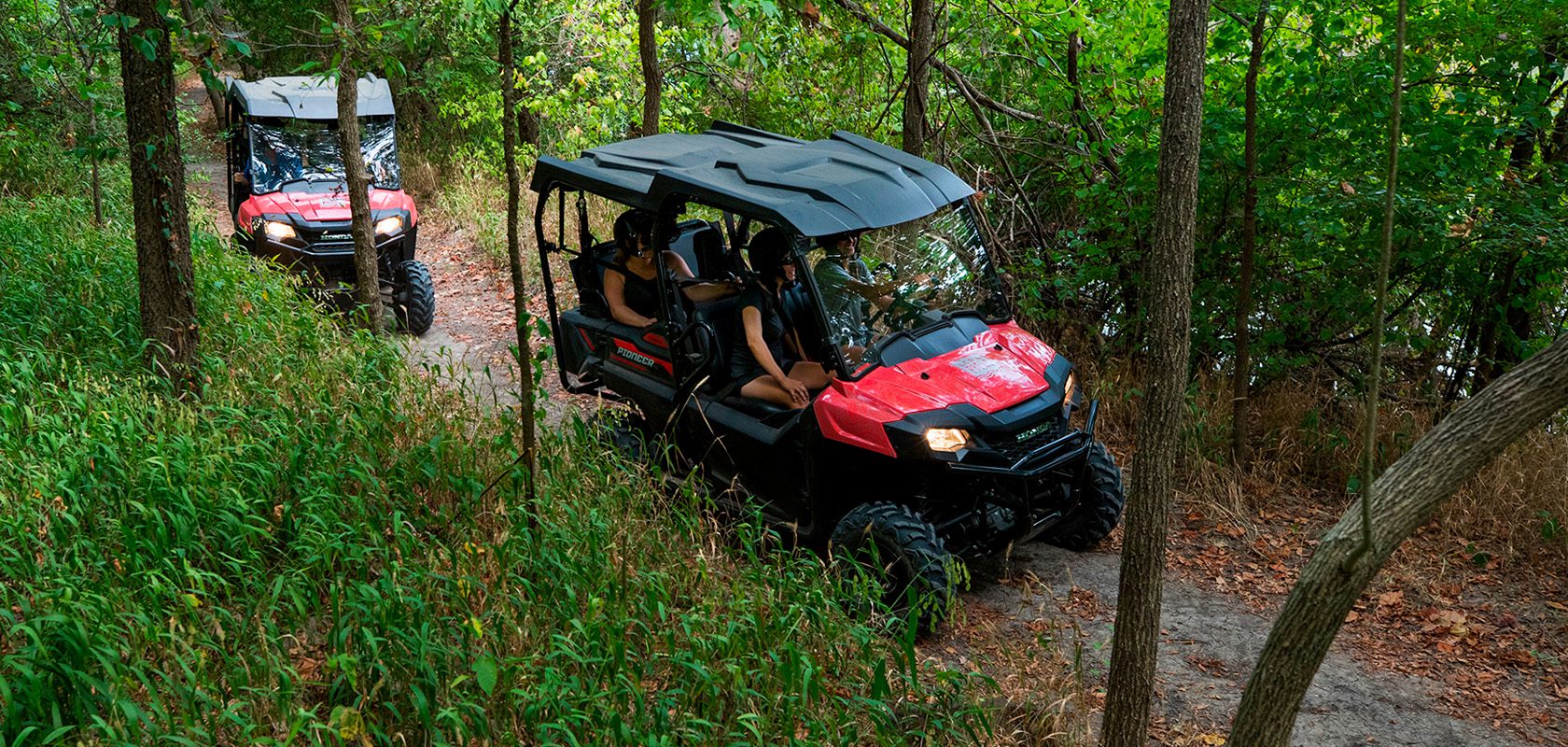This detailed color photograph captures two red ATV vehicles navigating a dirt path through dense, green, and brown woodland filled with heavy vegetation and trees. Both vehicles, resembling large off-road carts with open sides, black plastic roofs, and rubber wheels, are coming toward the bottom right of the image. The leading ATV, equipped with a windshield and lights, seats four occupants who are strapped in and wearing helmets. While it is not clear if the trailing ATV is also occupied, it mirrors the design and structure of the front vehicle. The scene evokes a sense of adventure, suggesting the passengers might be embarking on a safari, an excursion, or a leisurely drive through the forest.